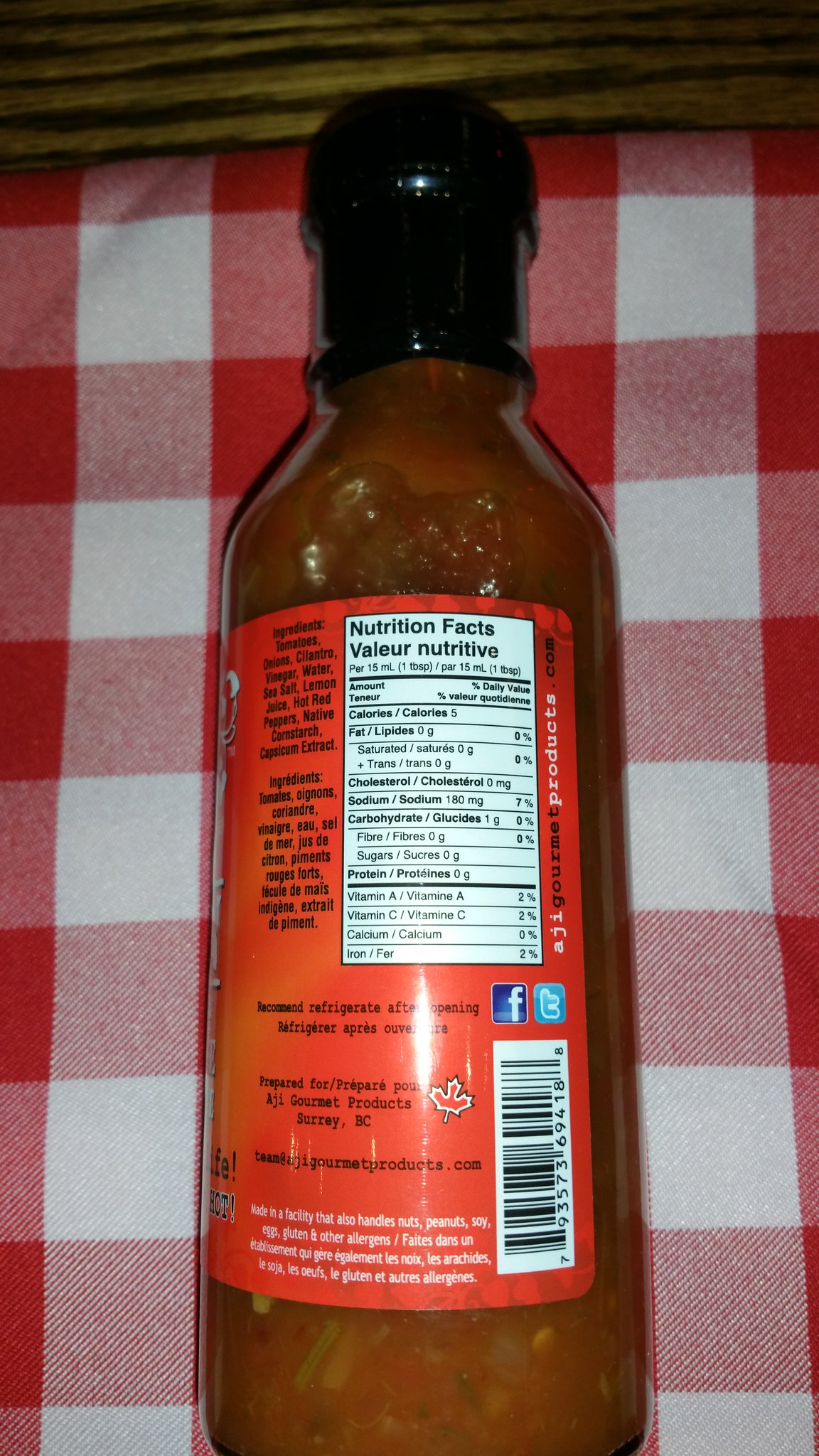An aerial overview showcases a vertical image with a limited background. The focal point is a meticulously woven structure of brown sticks, resembling a handcrafted basket. Resting at the bottom of the basket is a piece of cloth featuring a white and red checkered pattern, reminiscent of a cozy picnic blanket. Placed atop the cloth is a bottle with a black lid, containing a brownish-red liquid interspersed with chunks of various vegetables. The bottle's red label displays nutrition facts and a barcode, adding a touch of modernity to the rustic scene.